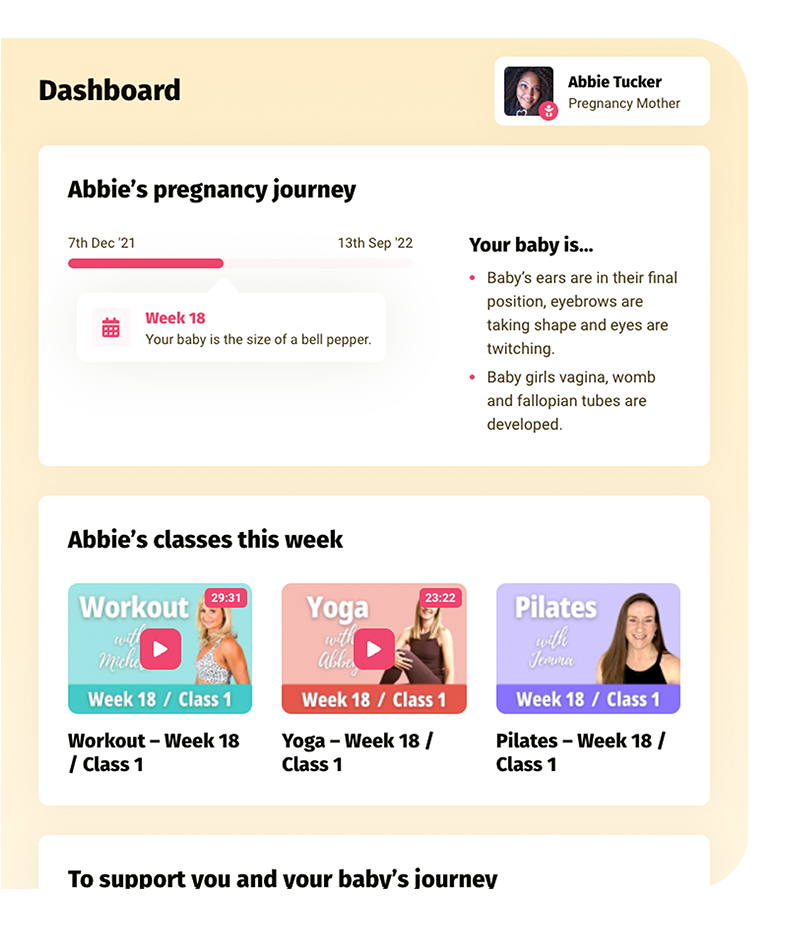This image showcases a pregnancy tracking dashboard designed to monitor Abby Tucker's pregnancy journey. 

The dashboard features a light tan background with the word "DASHBOARD" prominently displayed in black bold font in the upper left-hand corner. In the top section, a white block displays the name "Abby Tucker" alongside a profile picture of a woman with black hair. Below Abby's name, the label "Pregnancy Mother" is indicated.

Further down, another block titled "Abby's Pregnancy Journey" is visible. Beneath this title, a timeline is presented, classified with two key dates: "7th December 21st" at the beginning and "13th September 22" at the end. A red status bar stretches from the start to approximately the middle of the timeline, indicating the current date within the pregnancy period.

Below the timeline, the dashboard details that Abby is at "week 18" of her pregnancy, with an added note that her baby is "the size of a bell pepper." To the right, a section elaborates on the baby's development at this stage, specifying that "baby hairs are in their final position," "eyebrows are taking shape," and "eyes are twerking."